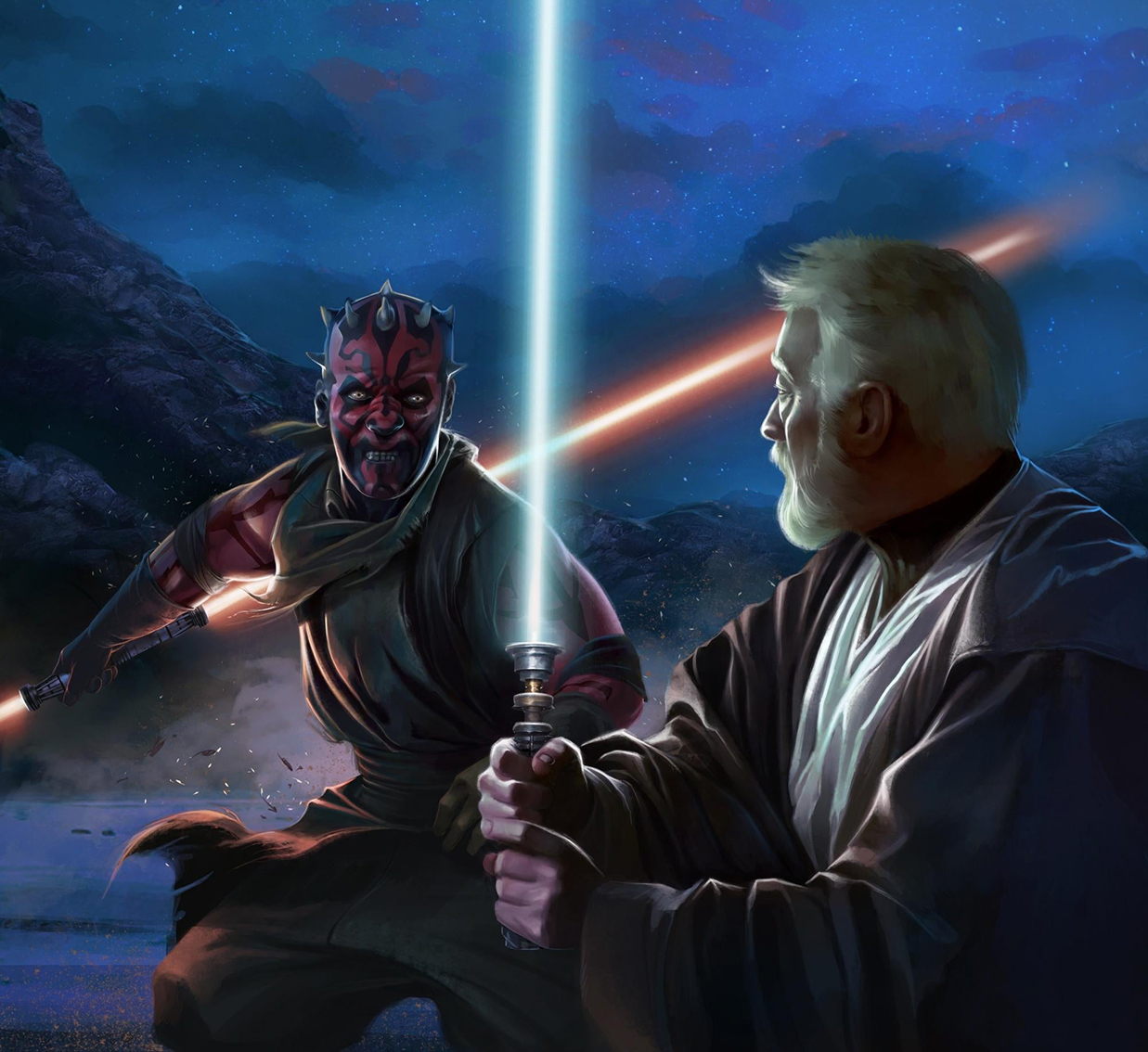This scene is a detailed, digital fan art resembling a Star Wars movie frame in a cartoonish style. The backdrop is a dark, blue-hued environment, with rocky mountains also bathed in shades of blue, under a sky that's teeming with stars, adding an extraterrestrial ambiance. The landscape appears almost desert-like, possibly just after dusk, with faint traces of purple and pink blending into the royal blue sky.

In the foreground, on a flat, blue surface, stand two iconic characters in a dramatic face-off. On the left, is Darth Maul, recognizable by his red and black demon-like face adorned with multiple small horns. His eyes are striking, with black dots in stark white. Clad in a combination of red and black clothing, he wields a double-sided red lightsaber that emits a threatening glow from both ends of the handle.

Facing him, slightly closer to the viewer, is a Jedi with a distinguished appearance. He has gray hair and a matching gray beard, and is wearing a layered outfit featuring a dark brown robe over a grayish-brown puffy shirt. His blue lightsaber, glowing intensely, is held firmly with both hands. The Jedi's determined expression and combat-ready stance indicate that a duel is imminent.

The vivid contrast of their lightsabers against the darker background, along with the intricate details of their attire and expressions, heightens the sense of tension and anticipation in this meticulously crafted scene.